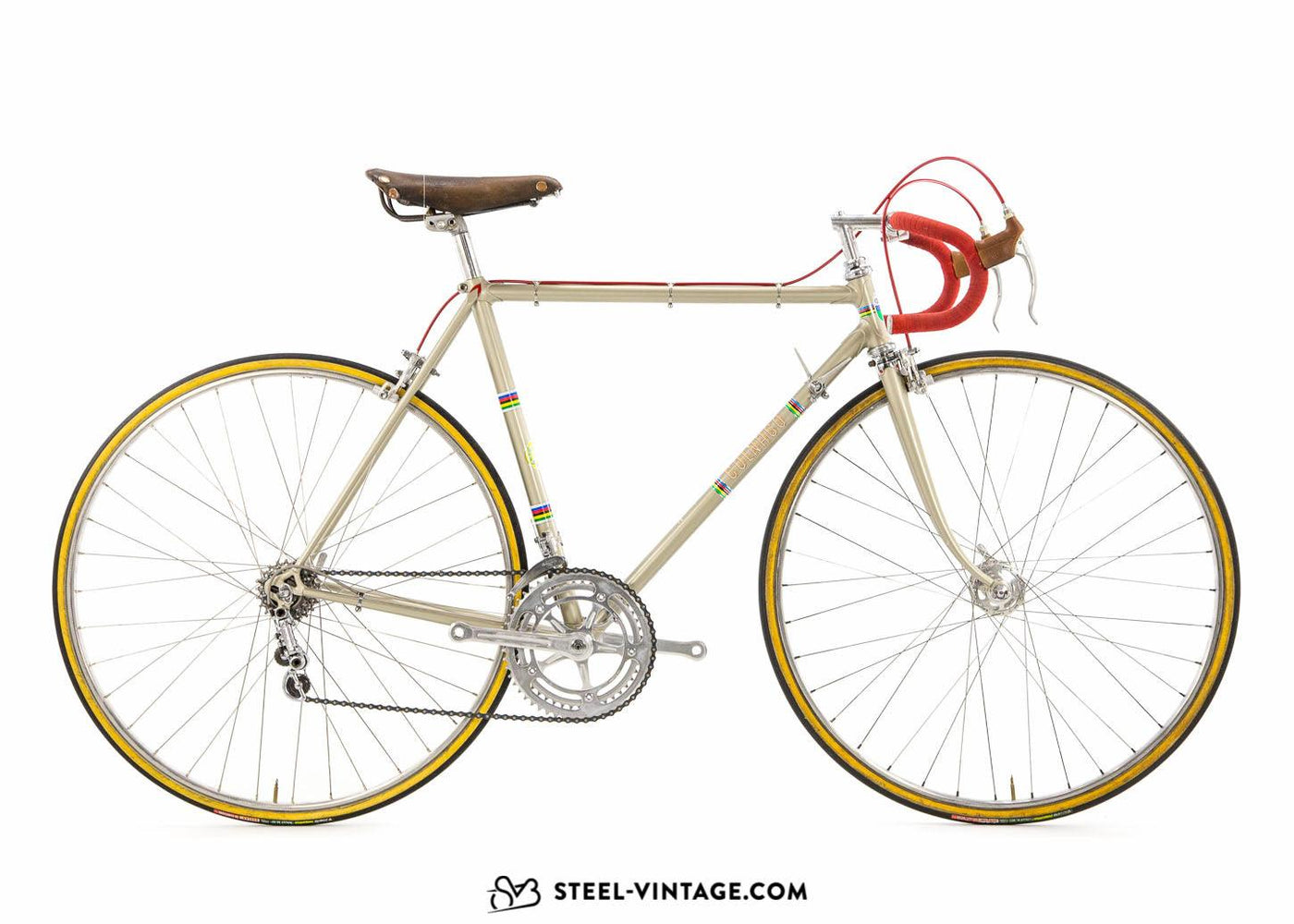This photograph showcases a vintage 10-speed bicycle positioned side-on and facing to the right. The bike features a clean, white frame complemented by a sleek black seat. The wheels display a striking combination of a dark charcoal gray outer rim with a golden inner rim, contributing to its old-fashioned charm. Noticeable are the numerous spokes leading to the hub, clearly visible and defining the wheel structure. The gear system and chain link to a rear derailleur, but the bike lacks pedals, exposing just the cranks. The handlebars are a vibrant red and curve downwards, complete with silver brake handles and corresponding brake wires—red towards the rear brake and regular wires to the front brake. Accentuating its classic vibe, the bicycle bears the inscription "STEEL VINTAGE DOT COM" in black letters underneath. Despite some conflicting descriptions about the frame color, the overall presentation of the bike underscores its vintage appeal, making it a definitive street bike rather than a modern, high-tech or mountain model.